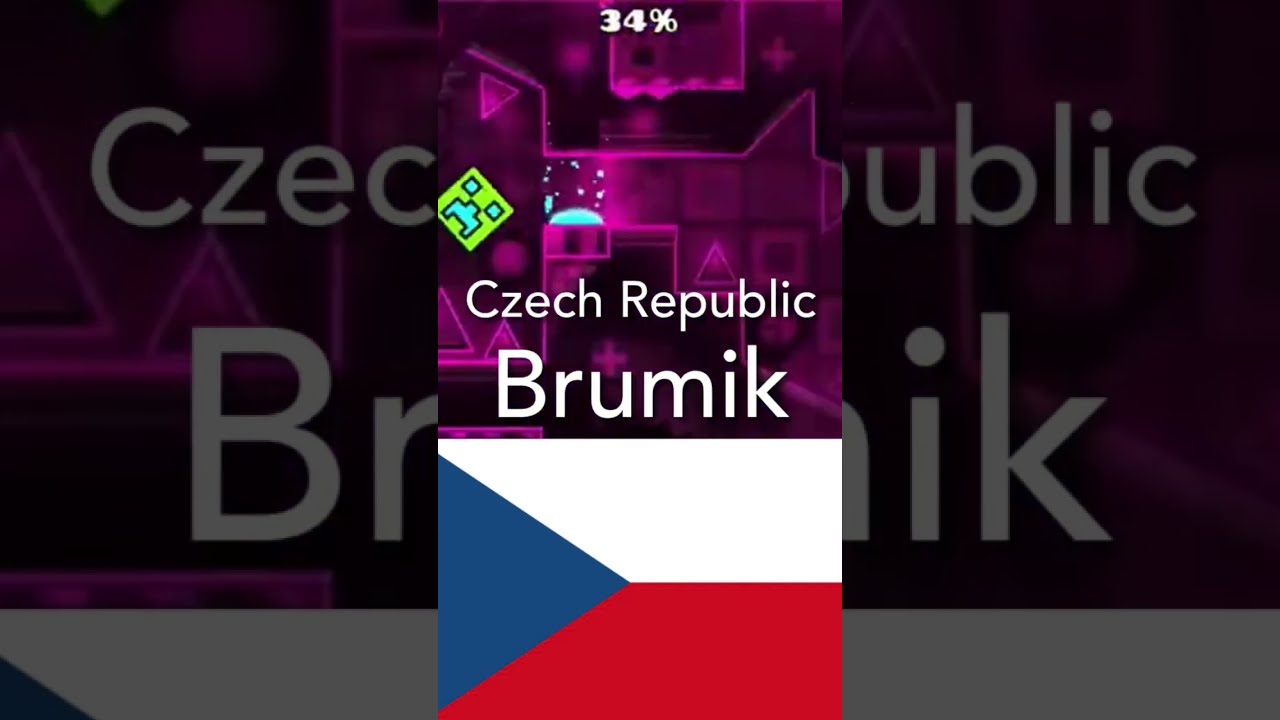The image consists of three panels, with a central panel flanked by two underexposed, darker panels. The central panel is brightly lit and clearly shows a flag of the Czech Republic at the bottom, characterized by a blue triangle on the left and horizontal white and red stripes. Superimposed in the center of this panel are the words "Czech Republic Brumik." Above the flag, the background features creative and interesting purple tunnels and tubes, with some geometric shapes including triangles. There's also blue fire emerging from one of the tubes and a small frowny emoji off to the left. At the very top of the image, the text "34%" is displayed in white. The left and right panels appear to be blow-ups of the left and right sections of the central panel, but they are darker and less focused, serving as large borders for the main image.